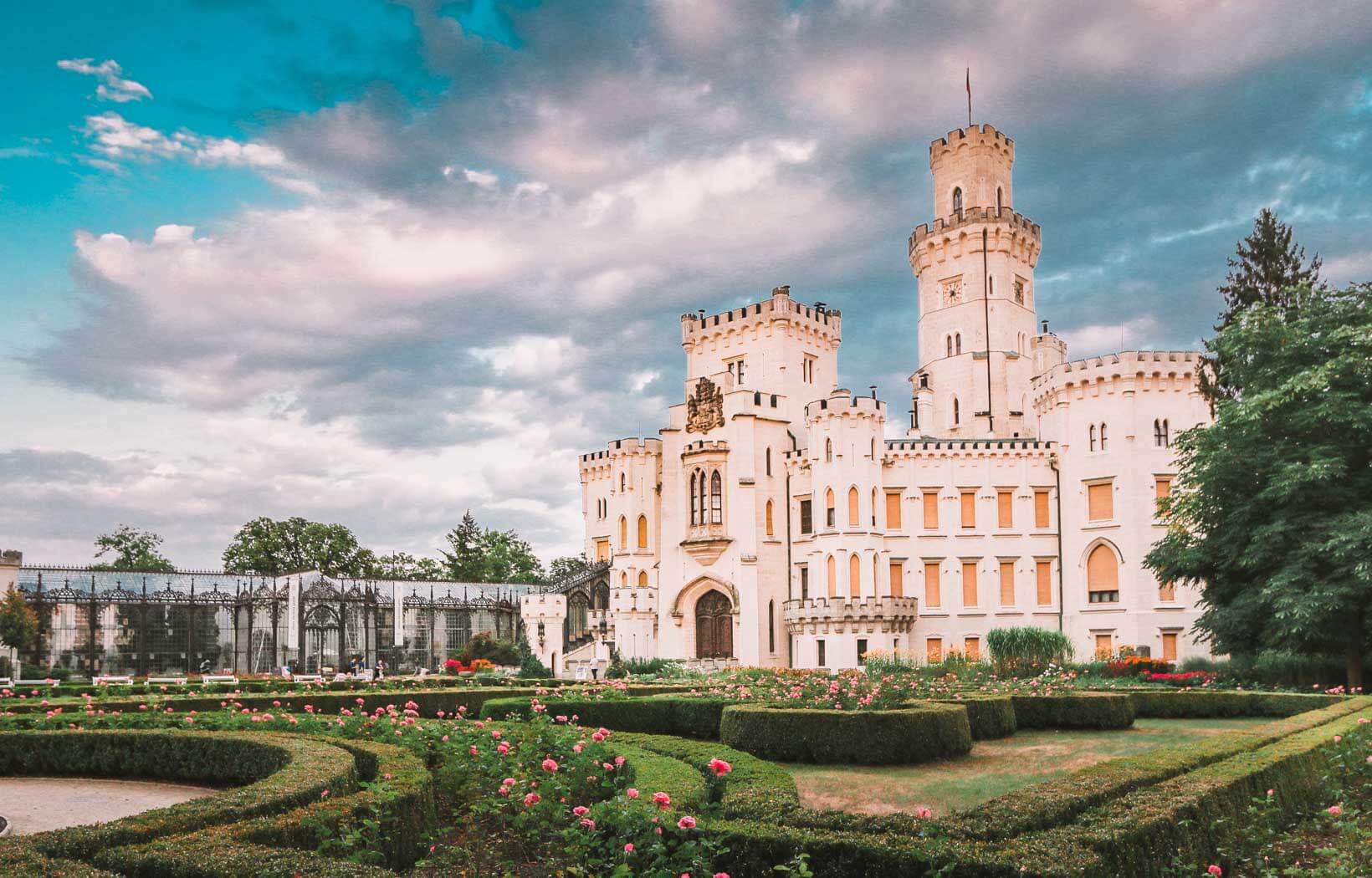The image depicts a professional piece of artwork that is indistinguishable from a high-quality photograph due to its detailed and pristine appearance. The centerpiece of the composition is a grand, bone-white palace with yellow and brown accents, and a prominent brown front door. This stately building, which could be a mansion, castle, or palace, appears to be a historical site potentially open for public tours. 

Surrounding the palace is a beautifully manicured garden. To the left, there is a white building with black trim, likely serving as a greenhouse with clear windows revealing various plants inside. To the right stands a huge, lush green tree. The garden features perfectly trimmed hedges and vibrant flowers, including pink, red, and orange blooms, contributing to the palette of green from the foliage. The lawn area presents a mix of green and yellow hues, with the bushes arranged in intricate patterns resembling mazes or circles, some adorned with pink flowers in the middle. The sky above is a mix of blue with scattered white and gray clouds. No people are visible on the grounds, and the image contains no text, focusing entirely on the serene and majestic scene.